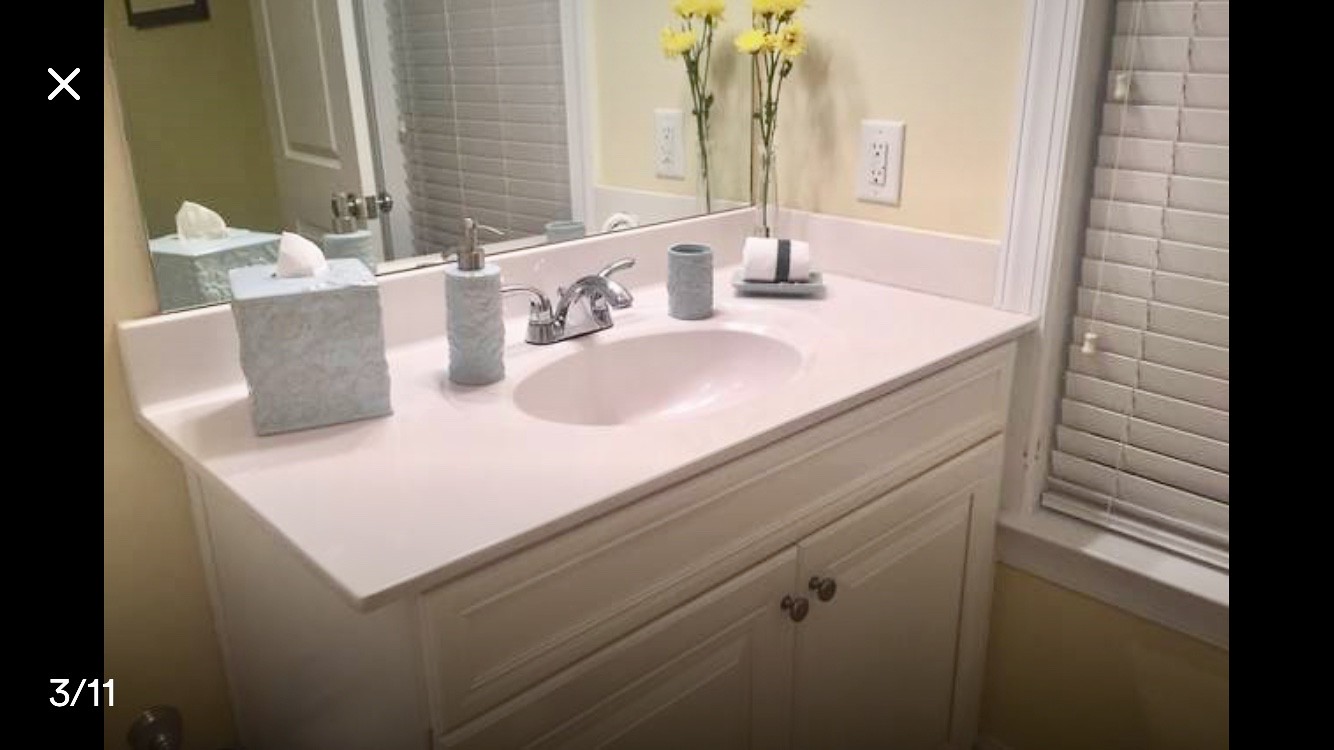The photograph captures an indoor bathroom setting in landscape orientation. The focal point is a modern sink and its surrounding elements. The sink is situated on a countertop that appears to be either white or a very light pink, complemented by an oval-shaped basin. The countertop, which occupies the center of the image, is framed by cabinets below and various decorative items above.

On the right side of the sink, there is a clear glass vase containing yellow flowers, adding a cheerful touch to the scene. Adjacent to the vase is a shallow gray dish, housing a rolled-up white cloth with a black stripe, suggesting an aesthetic and functional accent. Near the upper right edge of the sink countertop stands a light blue-green cup, while a matching soap dispenser with a sleek chrome pump is positioned on the left edge. To its left, a square tissue box, in the same light blue-green hue, holds a white facial tissue emerging from the top.

Beneath the countertop are white cabinet doors, each fitted with dark metal handles, providing a crisp contrast to the cabinetry. The right side of the room reveals a pale yellow wall hosting an electrical outlet with two vertically arranged plugs. In the far-right background, a window with white blinds fully drawn down sits within a white frame, allowing controlled lighting into the room.

Enhancing the scene's coherence, the sink features a chrome faucet with a gentle curve, flanked by two curved metal handles for hot and cold water control. This detailed composition combines functionality with subtle elegance, presenting a neatly organized and tastefully decorated bathroom space.